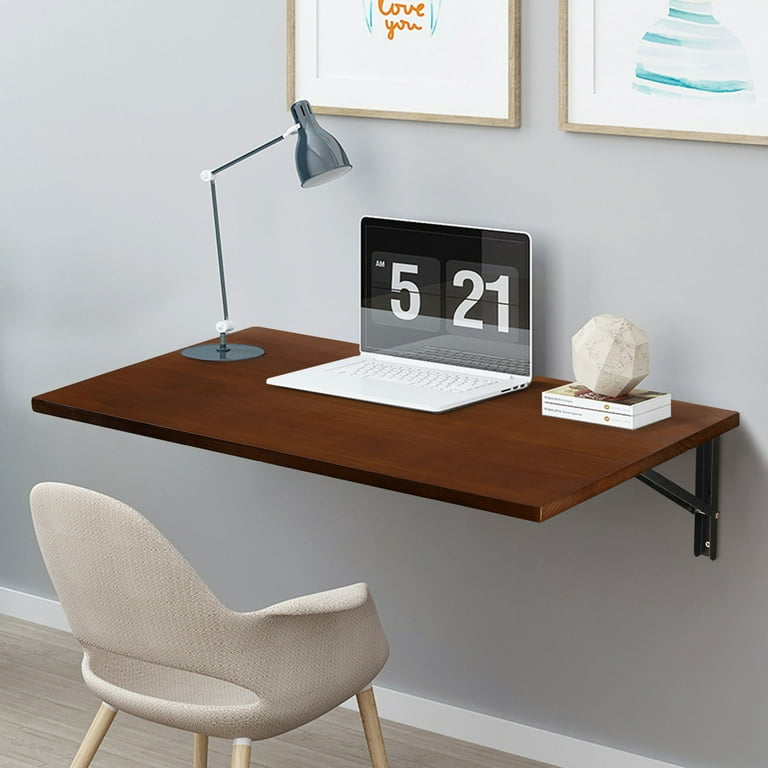The image depicts a modern, minimalist workspace. Central to the scene is a dark brown, wall-mounted floating desk with no legs, supported by black brackets. On the left side of the desk sits a sleek silver-gray desk lamp with white hinges, resembling the iconic Pixar lamp. Positioned at the center of the desk is a white laptop displaying "5:21 AM" in large white letters on a black and gray background. To the right of the laptop are two stacked books, topped with a spherical marble-like decorative object. A white chair with light brown wooden legs is placed in front of the desk, resting on a light gray, laminated floor. The backdrop of this workspace is a light gray wall adorned with two paintings in very light brown frames. The left painting bears the text "Love you" in orange cursive, while the right painting displays blue and white stripes, both extending off the edge of the image. The overall aesthetic is clean, functional, and subtly artistic.